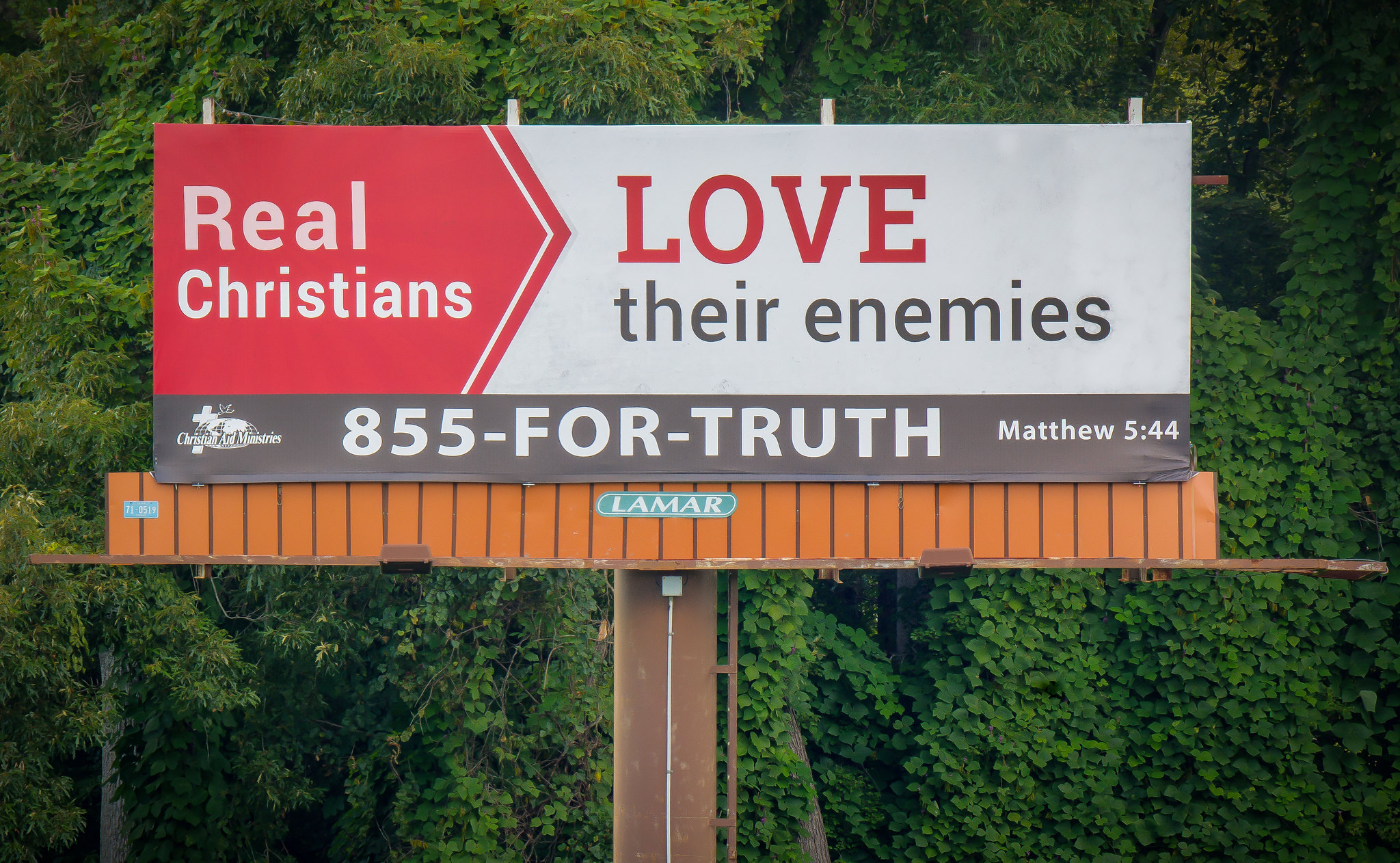The image features a horizontal billboard set against a backdrop of lush, green trees and bushes covered in kudzu. The billboard, mounted on a sturdy brown metal pole, is rectangular in shape. The left side of the billboard has a striking red background in the shape of an arrow pointing right, emblazoned with the words "Real Christians" in white text. The right side features a white background with the word "Love" prominently displayed in large red letters, followed by "their enemies" in smaller black text beneath it.

At the bottom of the billboard, there is a grey strip bearing additional information: on the left, it says "Christian Ministries" along with a logo featuring a cross; in the middle, a telephone number formatted as 855-4-TRUTH; and on the right, the biblical reference Matthew 5:44. 

The base of the billboard indicates it is supported by Lamar, with a blue emblem and a brownish base. The greenery in the background enhances the contrast and detail of the billboard's message.